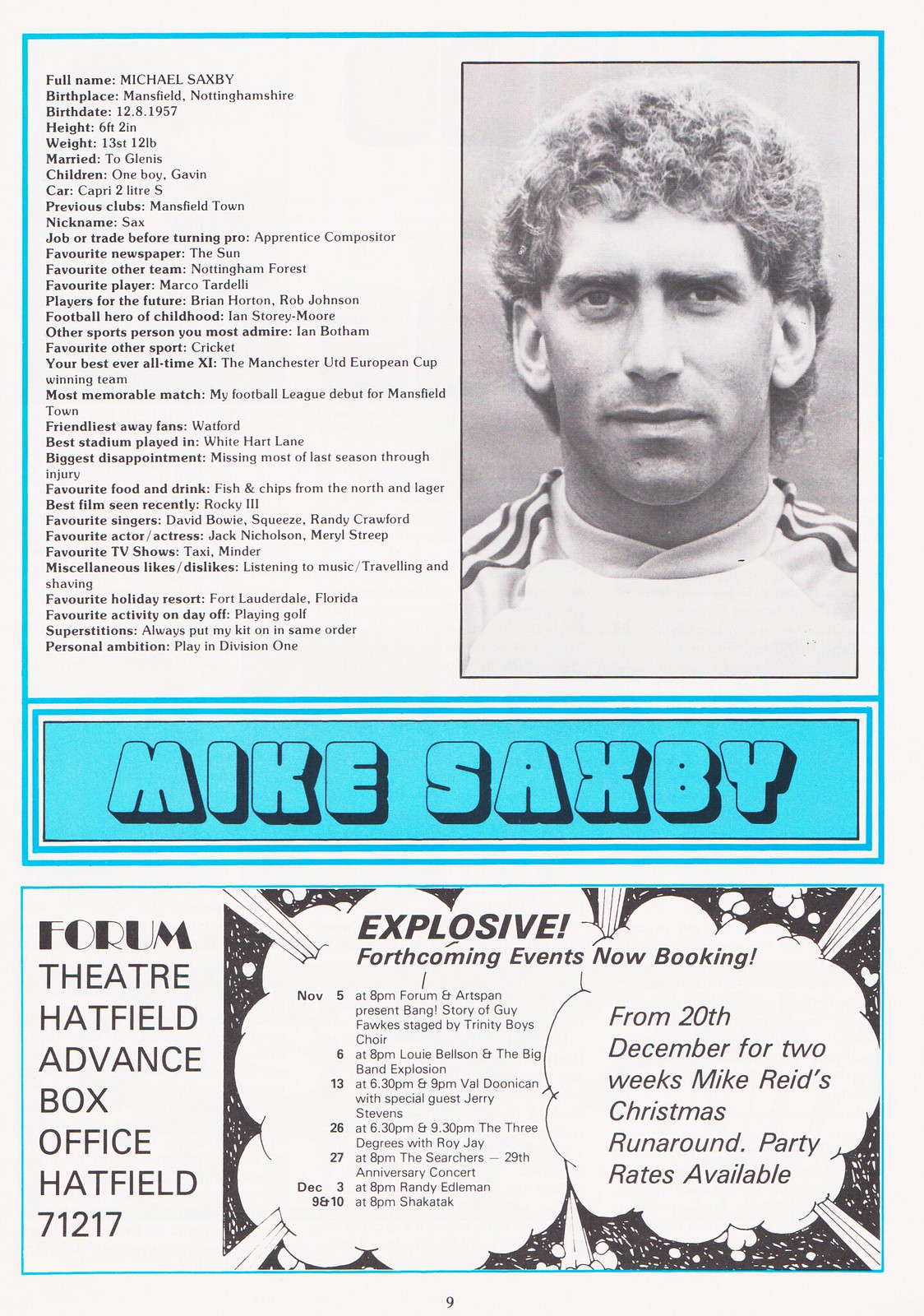This is a detailed poster image featuring a black-and-white photograph of a man, identified as Mike Saxby, a soccer player, positioned at the top right side. Saxby, who is wearing a soccer uniform with a striped design on the shoulders, stares directly into the camera. The photograph is rectangular and the entire image has an overall bold and sporty aesthetic. On the left side, detailed textual information about Saxby is written in black, covering personal interests such as his favorite newspaper, team, player, and other sports, with cricket being a favorite. Below this section, against a blue background framed in black, the name "Mike Saxby" is prominently displayed in bold blue letters. Additional text at the lower left gives venue information, listing "Forum Theater, Hatfield, Advanced Box Office, Hatfield, 71217." To the right are two cloud shapes containing further descriptive text. The poster is evidently designed to highlight Saxby’s personality and achievements, blending personal trivia with promotional content.